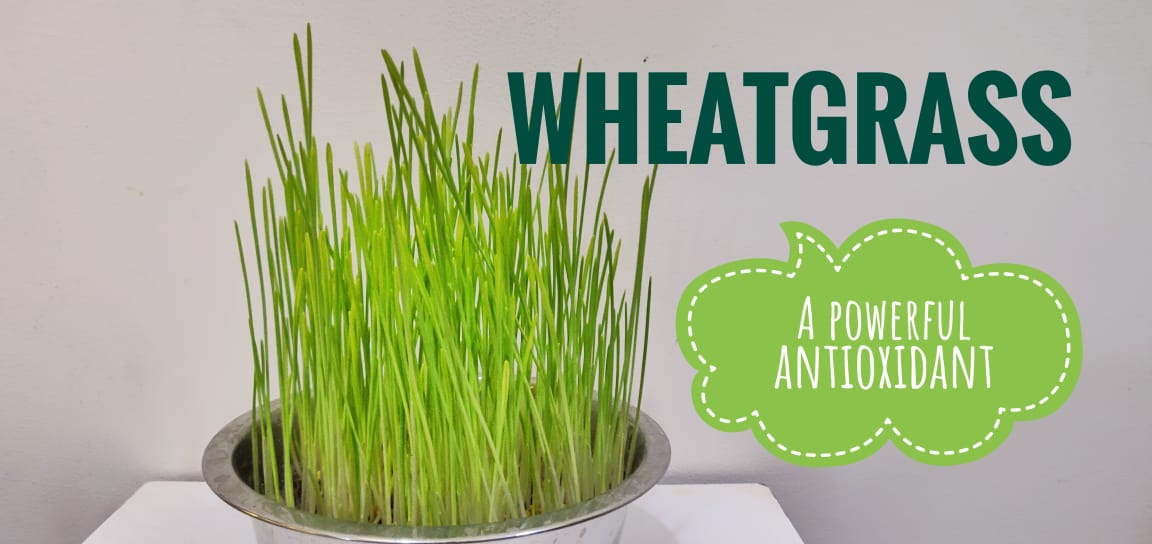The image shows a detailed and visually appealing advertisement for wheatgrass. At the center, a lush, vibrant crop of wheatgrass grows straight up from a sleek, metallic silver bowl. The grass transitions from a lighter, almost whitish green at the base to a rich, darker green at the tips, reaching heights of six to seven inches. This verdant display is set on a clean, white table, which appears to be a small side table rather than a kitchen table. The backdrop features a dull, gray wall that enhances the vivid green hues of the wheatgrass.

At the top of the image, the word "WHEATGRASS" is prominently displayed in a deep, forest green font. Below this title, a bright, neon green speech bubble with a dotted white border and white font declares the plant's benefits, "a powerful antioxidant." This graphic blends seamlessly with the photograph, emphasizing both the health benefits and the aesthetic appeal of the wheatgrass.